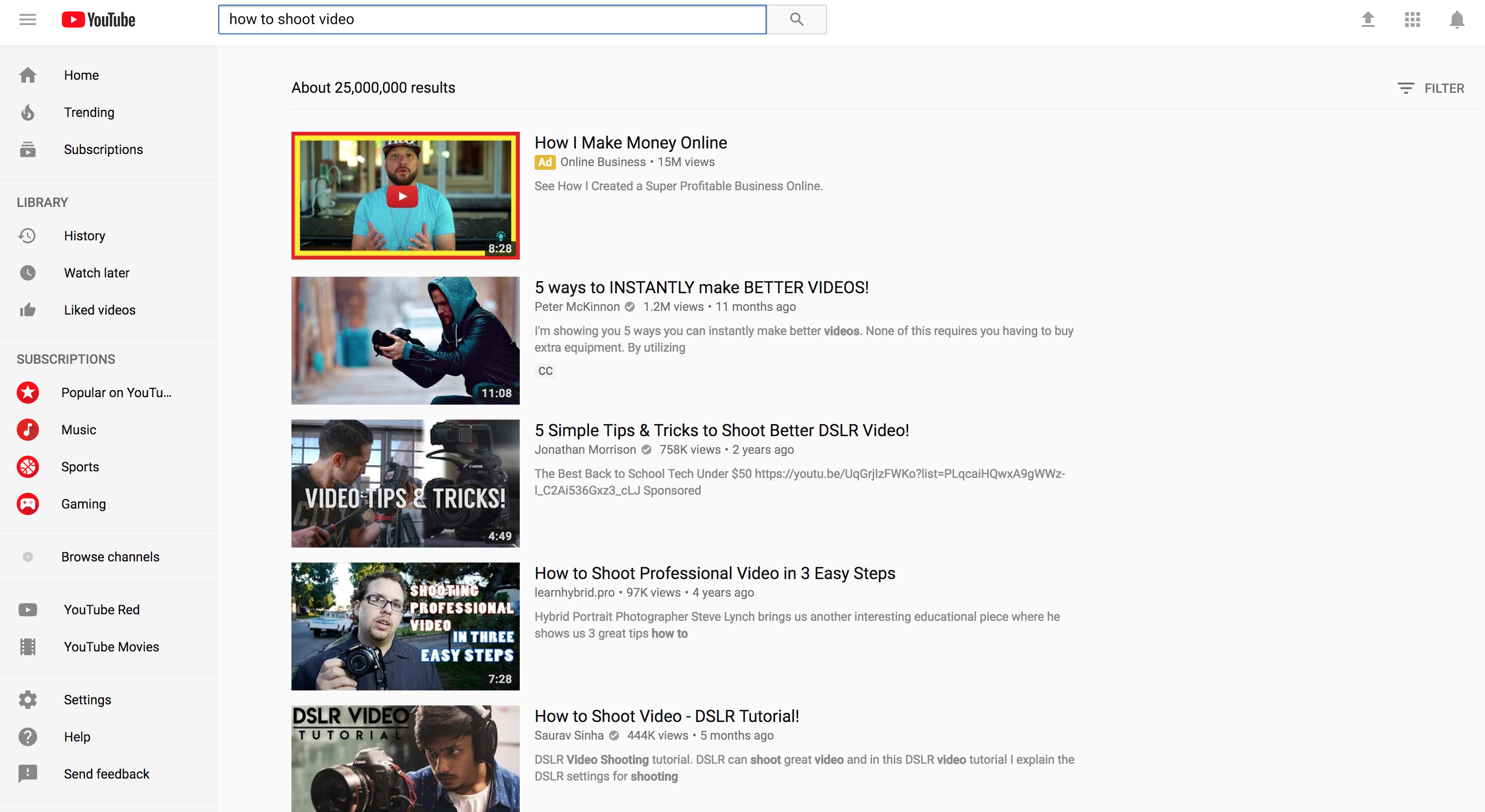In the upper left corner of the image, there are three lines indicating a pull-down or pop-out menu, commonly associated with YouTube. The menu items listed include: Home, Trending, Subscriptions, Library, History, Watch Later, Videos Liked, Subscriptions, Popular on YouTube, Music, Sports, Gaming, Browse Channels, YouTube Red, YouTube Movies, Settings, Help, and Send Feedback.

At the top of the screen, the search bar contains the phrase "how to shoot videos," resulting in about 25 million search results. Below this, there are five video thumbnails, each accompanied by detailed descriptions.

1. The first video is an advertisement titled "How I Make Money Online," boasting 15 million views. The description highlights strategies to create a profitable online business.
   
2. The second video, "Five Ways to Instantly Make Better Videos" by Peter McKinnon, has 1.2 million views and was uploaded 11 months ago. Peter demonstrates five techniques to enhance video quality without purchasing additional equipment.

3. The third video, "Five Simple Tips to Shoot Better DSLR Video," created by Jonathan Morrison, has garnered 758,000 views over the course of two years. It promises straightforward tips for improving DSLR video footage.

4. The fourth video focuses on affordable tech with the title "The Best Back to School Tech Under $50."

5. The fifth video, "How to Shoot Professional Videos in Three Easy Steps" by Learn Hybrid Pro, offers a straightforward guide to achieving high-quality video production.

The detailed layout and the comprehensive descriptions provide a clear snapshot of YouTube’s interface and the content available pertaining to video shooting techniques.